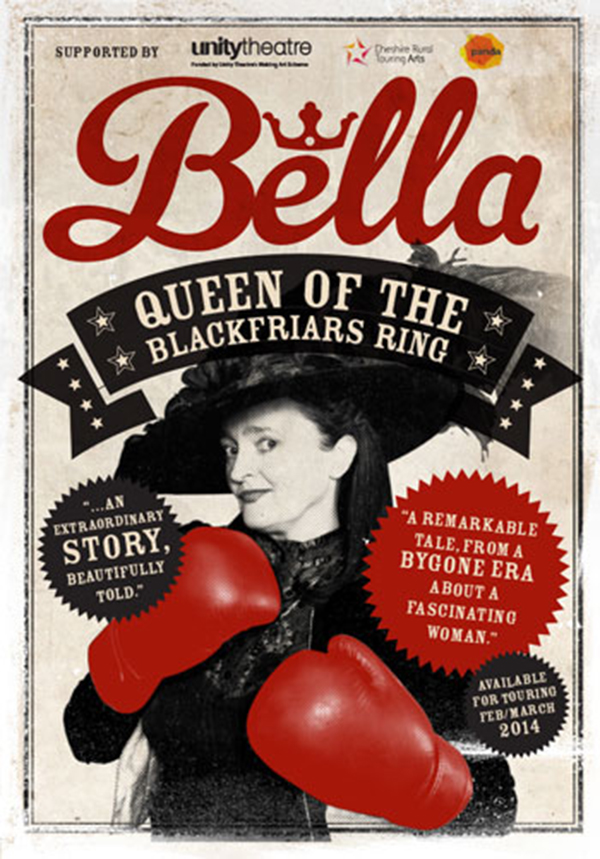The image depicts a vintage-style theater poster promoting a dramatic play titled "Bella." The poster features a monochromatic palette accented with striking red details. The title "B-E-L-L-A" is elegantly written in bold red cursive script, with a regal crown adorning the lowercase "e." Below the title, there's a black ribbon-like banner with white text declaring "Queen of the Blackfriars Ring."

At the center of the poster, there's a black and white photograph of a white woman from a bygone era, possibly Victorian. She has dark hair and wears a top hat and a traditional, long black outfit. In a stark contrast to the monochrome theme, she dons a pair of bright red boxing gloves, her expression one of mild surprise.

Surrounding the image, several circles provide critical accolades and additional information. One black circle states, "An extraordinary story beautifully told," while a red circle highlights, "A remarkable tale from a bygone era about a fascinating woman." A smaller circle at the bottom announces the availability of the show for touring in "February/March 2014."

The background of the poster is primarily white, and at the very top, it notes support from the Unity Theater. This detailed and visually compelling advertisement captures the essence and intrigue of the theatrical production it promotes.